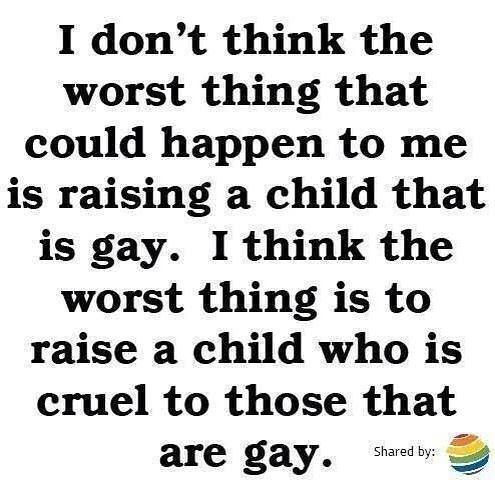The image features a poignant, motivational quote presented over a stark white background with no borders or additional design elements. The text, typed in black ink using either a computer or typewriter, reads: "I don't think the worst thing that could happen to me is raising a child that is gay. I think the worst thing is to raise a child who is cruel to those that are gay." The quote is spread across nine lines, emphasizing thoughtful reflection. Near the bottom right corner, there's a small, vibrant symbol resembling a striped, glowing ball with colors transitioning from deep red, through orange, yellow, green, light blue, and dark blue. This symbol indicates that the quote is shared, adding a touch of inclusivity and a hint of social media influence.